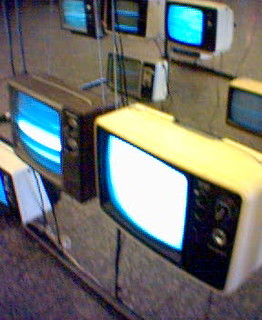The image depicts a captivating display of vintage cathode ray tube (CRT) televisions from previous generations, arranged in a somewhat chaotic yet intriguing manner. There are eight old-style tube TVs in total, all varying in size and color.

The two central TVs are the most prominent: one is encased in white plastic with black accents and features a blank white screen, while the other is brown wood-grain with a blue screen streaked with white bars. Both are supported by a complex metal contraption consisting of wires and rods.

Behind these primary televisions, five more sets are mounted, each held up by additional metal railings and wires. The TV immediately below the central units is another white plastic model, closely resembling the upper one with black dials and a blank screen. Additional sets include a mix of tan, silver, and white plastic casings, some showing blue and green hues or static on their screens.

This intricate setup is situated against a wall in a grayish-brown hue that contributes to the nostalgic ambiance. The ground below is covered with a rough industrial gray carpet, enhancing the sense of a bygone era. The image, though blurry and reminiscent of a low-resolution magazine ad or shop display from the 1980s or early 90s, presents an artistic and thought-provoking assembly of vintage technology.